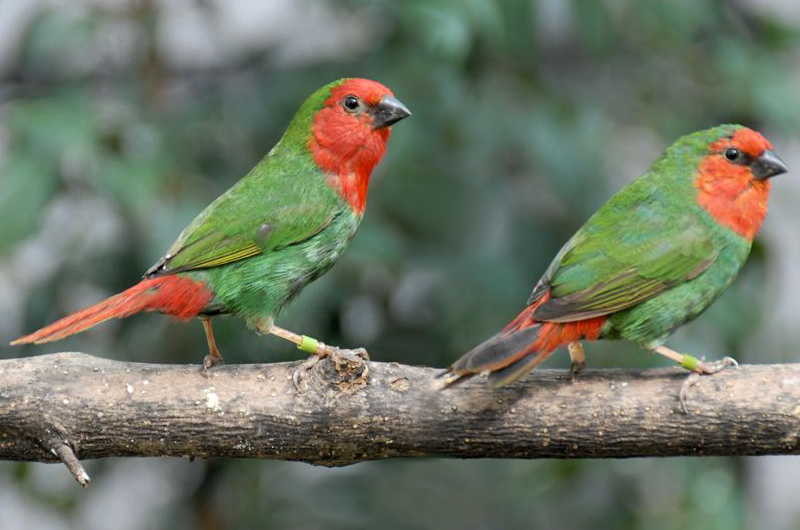This close-up photograph captures two nearly identical birds perched on a medium-sized tree branch. The background consists of muted, blurry shades of green and gray, hinting at forest foliage. Both birds are primarily green with vivid red faces extending from the tops of their heads to their necks, and sharp, small black beaks. Their large, round black eyes add a touch of intensity to their gaze. They also have reddish tails, with the bird on the right featuring more black at the tips of its feathers. These birds have yellowish-tan legs with delicate, gray claws, each sporting a small green band on one leg, possibly indicating they are being tracked. The bird on the right appears slightly shorter and chubbier, enhancing its endearing profile as it looks to the right.